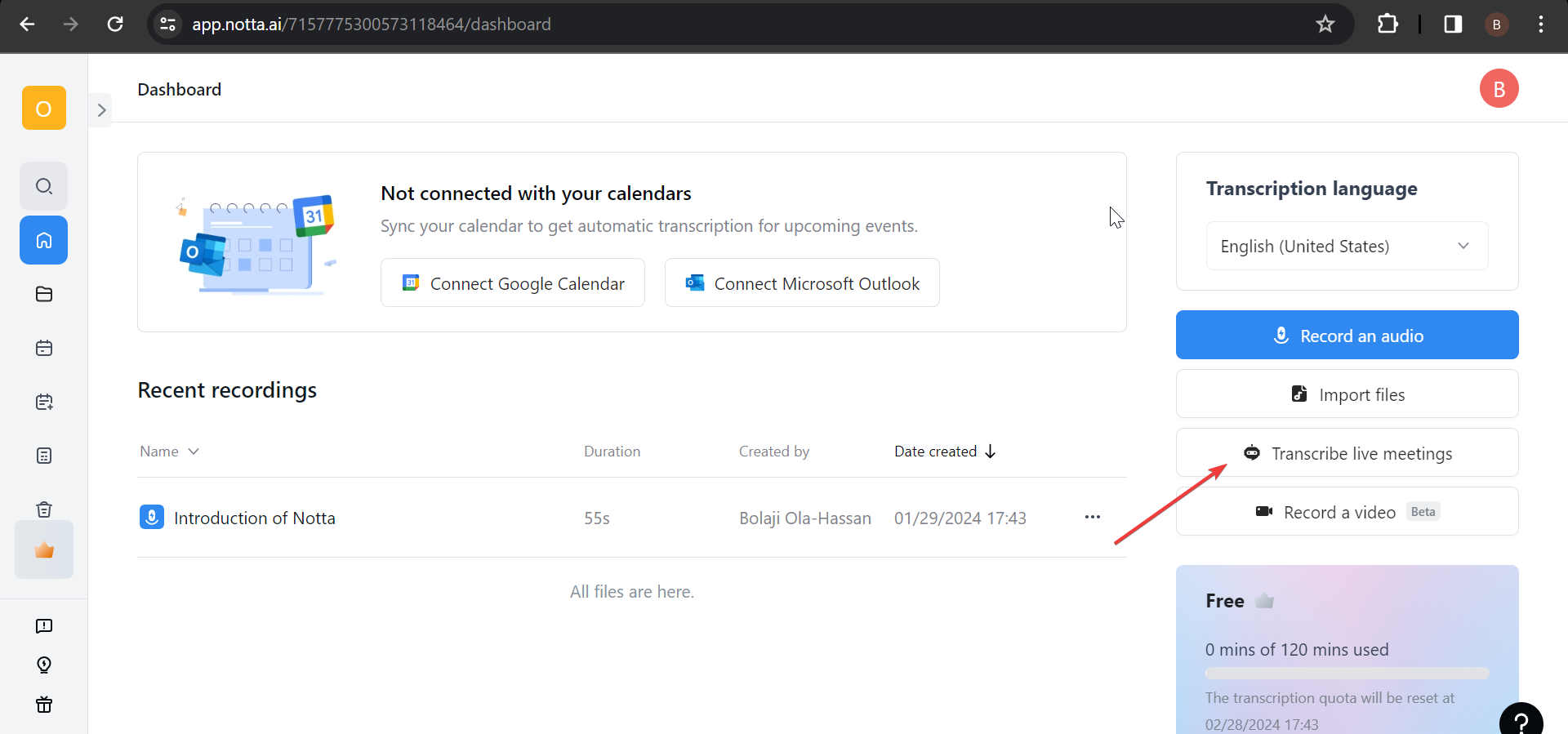Screenshot of a person’s web browser displaying the NATA AI web application dashboard. The browser's address bar reads "app.nata.ai/<series_of_numbers>/dashboard." The primary screen is mostly white and features a notification at the top that states, "Not connected with your calendars. Sync your calendar to get automatic transcriptions for upcoming events." Below this notification, there are two buttons: one for connecting to Google Calendar and the other for connecting to Microsoft Outlook.

Directly under the notification, the dashboard is divided into sections. The first section, titled "Recent Recordings," features a drop-down menu labeled "Name." Within this menu, a single audio file is listed. This file is indicated by a blue microphone icon and is named "Introduction of NATA." Details for this file include a duration of 55 seconds, created by Bolahi Ola Hassan on January 29th, 2024, at 17:43 hours.

To the right of this recording, a red arrow points upward towards a button labeled "Transcribe Live Meetings." Adjacent to this, information indicates that the transcription language is set to English.